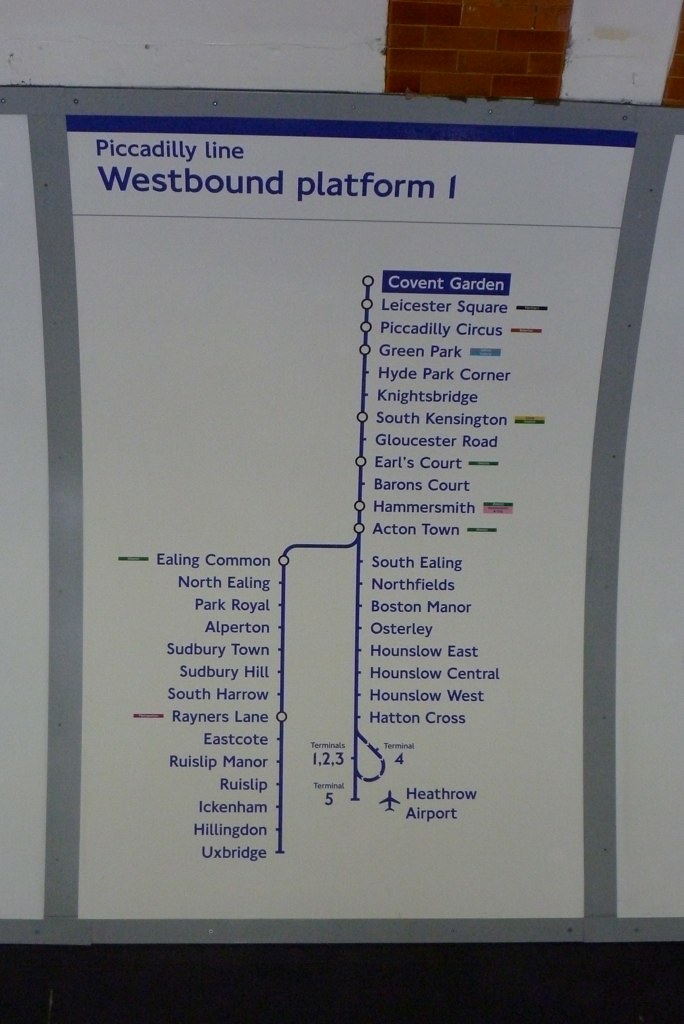This image captures a detailed sign on a white subway station wall, likely part of the London Underground's Piccadilly Line, given the references to familiar stops. The wall features sections of white and red brick, with the sign itself bordered by grey metal. At the top of the sign, there is a dark blue stripe followed by the text "Piccadilly Line" and "Westbound Platform 1" in blue. Below this, the sign shows a map with lines and dots indicating various stations, branching into two sections that list numerous stops. On the left column, stops include Ealing Common, North Ealing, Park Royal, Alperton, Sudbury Town, Sudbury Hill, South Harrow, Rayners Lane, Eastcote, Ruislip Manor, Ruislip, Ickenham, Hillingdon, and Uxbridge. The right column lists stops such as Covent Garden, Leicester Square, Piccadilly Circus, Green Park, Hyde Park Corner, Knightsbridge, South Kensington, Gloucester Road, Earl's Court, Barons Court, Hammersmith, Acton Town, South Ealing, Northfields, Boston Manor, Osterley, Hounslow East, Hounslow Central, Hounslow West, Hatton Cross, and Heathrow Airport, complete with station numbers and a curved line to emphasize connections.